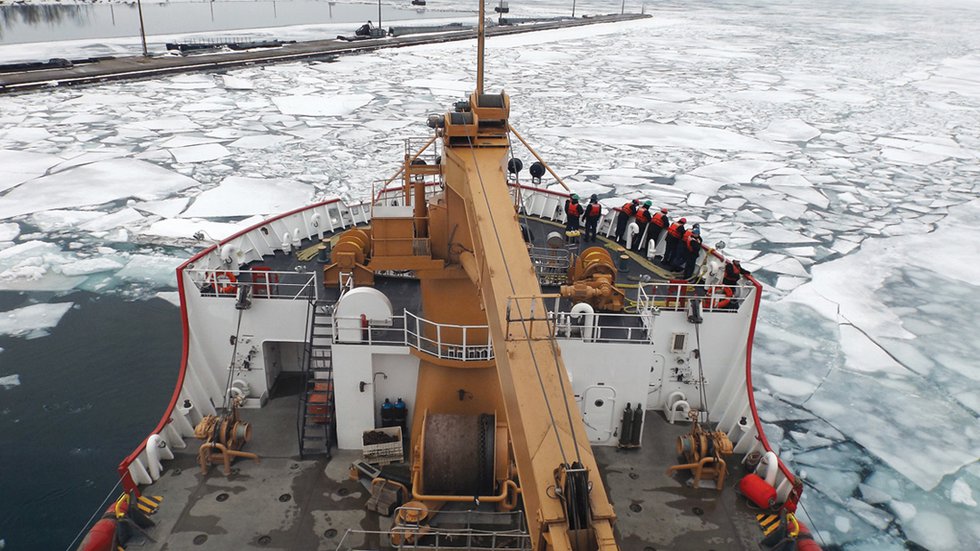In this detailed, daytime aerial view, a ship navigates through a sea of cracked, floating ice in what appears to be polar waters, potentially near the polar ice caps. The ship, which has a white exterior with a red border, features multiple levels — the second of which houses a number of people, identifiable by their orange or red vests and headwear. These individuals stand along the edge, looking out over the icy expanse below. The water is dark, contrasting sharply with the bright white ice chunks scattered across its surface. Mechanical objects and a door are visible on the boat, which offers stairs on its left side. Beyond the ship, a long, narrow structure resembling a sidewalk or median stretches into the distance, intersecting the icy landscape.